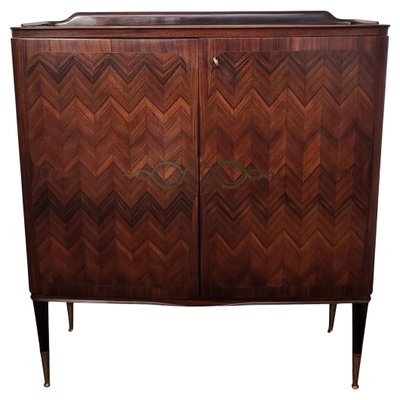The photograph depicts a vintage wooden cabinet with a dark finish, standing against an all-white background that obscures the floor, making the cabinet appear to float. The cabinet is slightly wider than it is tall, resembling a rectangular cube. It is elevated on four slender legs. The front of the cabinet features two doors adorned with a distinctive zigzag or chevron pattern in varying shades of wood, giving it a textured, dynamic appearance. Each door is fitted with large oval gold handles, each accompanied by smaller oval accents, adding a touch of elegance. At the top, a subtle lip suggests additional functionality, possibly hinting at a liftable feature. The overall look and feel of the piece suggest that it could be an old-timey radio player or a sophisticated bar unit.